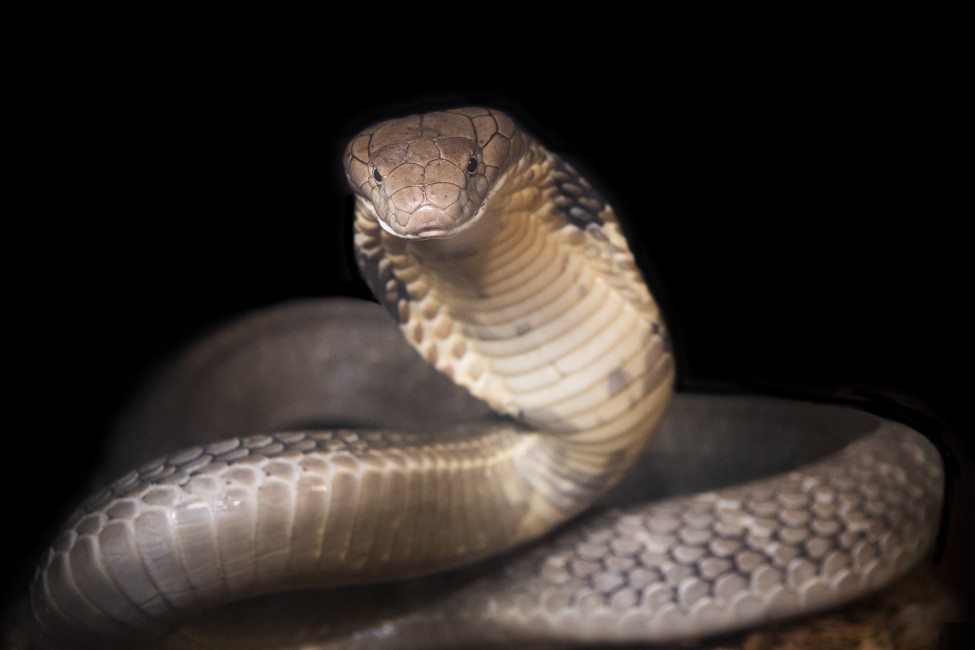This detailed close-up image captures a majestic cobra snake coiled against a stark black background. The spotlight highlights the snake's textured, medium gray scales and distinctive features. Its body coils extend gracefully across the frame, with the second coil disappearing towards the foreground, reflected on the shiny surface beneath. The snake's head is raised, giving a clear view of its flanged neck and the intricate lines along its ivory and beige underbelly. The head is marked by deep cracks and unique scales, complemented by intense black eyes that stare directly at the camera. The snake's poised stance and slightly upturned mouth suggest it is ready to strike, showcasing its regal and powerful presence.